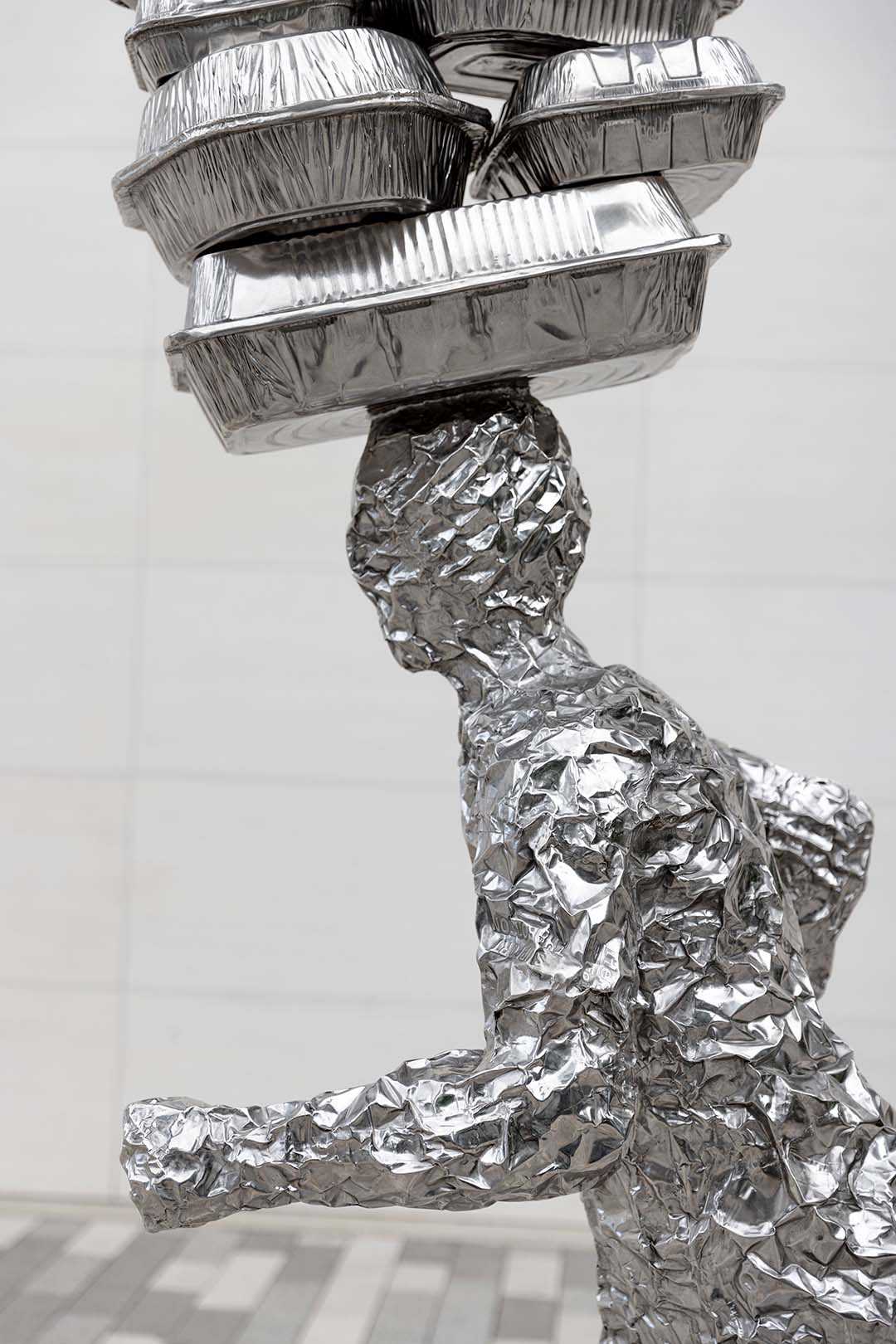This photograph showcases a creative sculpture of a human figure made entirely out of aluminum foil, set against a smooth white wall with a texture resembling large bricks. The floor beneath features a visually engaging checkered pattern in light gray, white, and dark gray tiles. The aluminum figure is depicted in mid-motion, with its right arm cocked behind and its left arm extended forward, suggesting a walking or running pose. Atop the figure's head, a precarious stack of disposable aluminum food containers, including rectangular and circular pans, rises impressively to the top edge of the image. This whimsical and intricate artwork captures attention with its detailed craftsmanship and playful balance of elements.